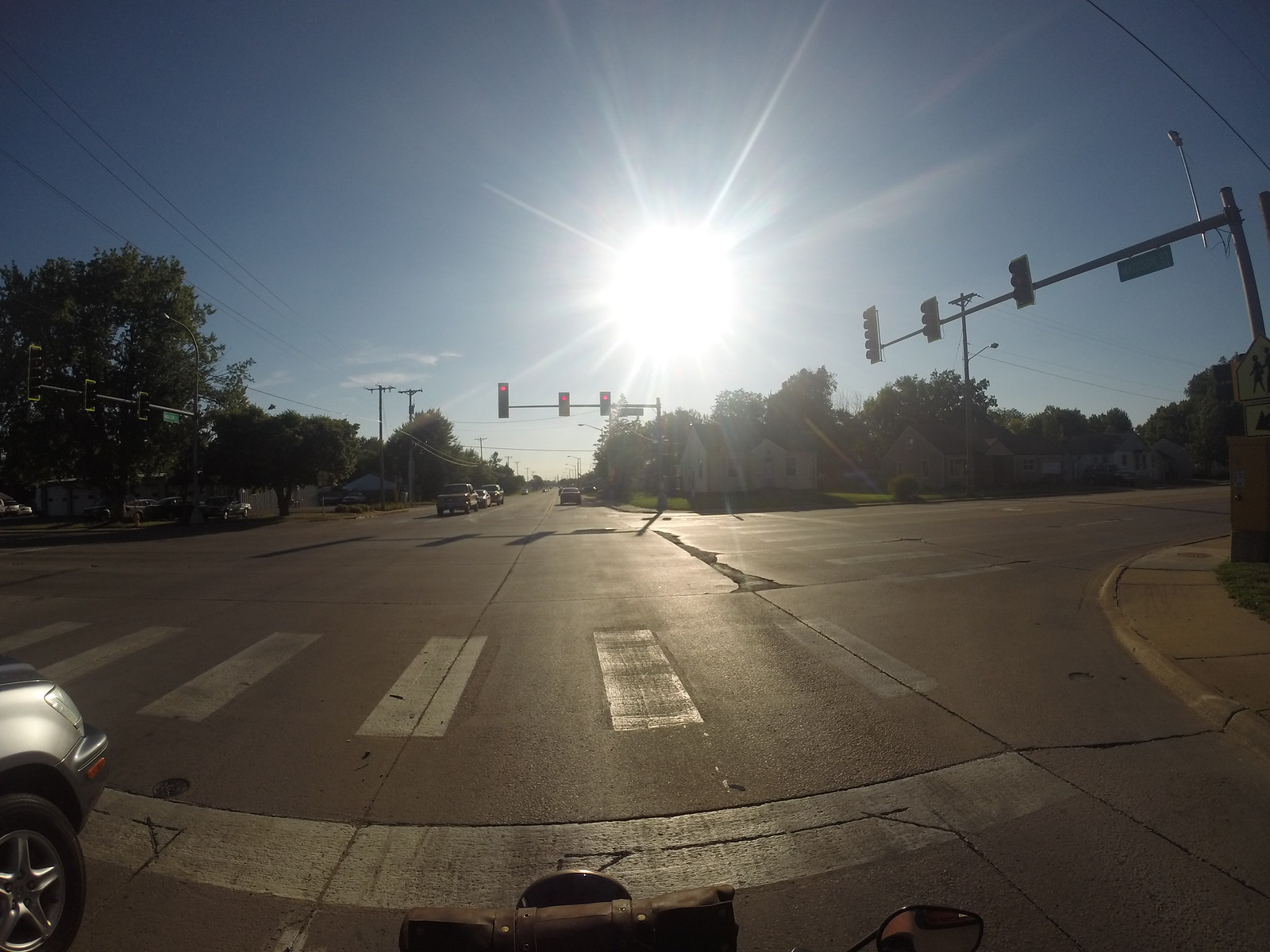This photograph captures a scene from the perspective of a vehicle, potentially a motorcycle, waiting at an intersection on a sunny day. The vehicle is facing directly into the bright, rising sun, casting a stark light across the image. A rearview mirror in the lower center suggests the vantage point might indeed be from a motorcycle. 

Ahead, a crosswalk spans the intersection, leading to a wide street that forms an X-shaped junction. In the lower left corner, a sliver of a silver car is visible, indicating nearby traffic. To the right of the intersection, streetlights stand tall, holding a trio of horizontal traffic lights currently glowing red. These traffic lights are affixed to a vertical pole at the intersection's edge.

On the far side of the intersection, other vehicles wait to turn, emphasizing the bustle of the crossing. Trees line the horizon, framing the scene with a touch of greenery. Above, the sky is a bright blue, dominated by the intense light of the sun, creating a vivid and starkly contrasting backdrop.